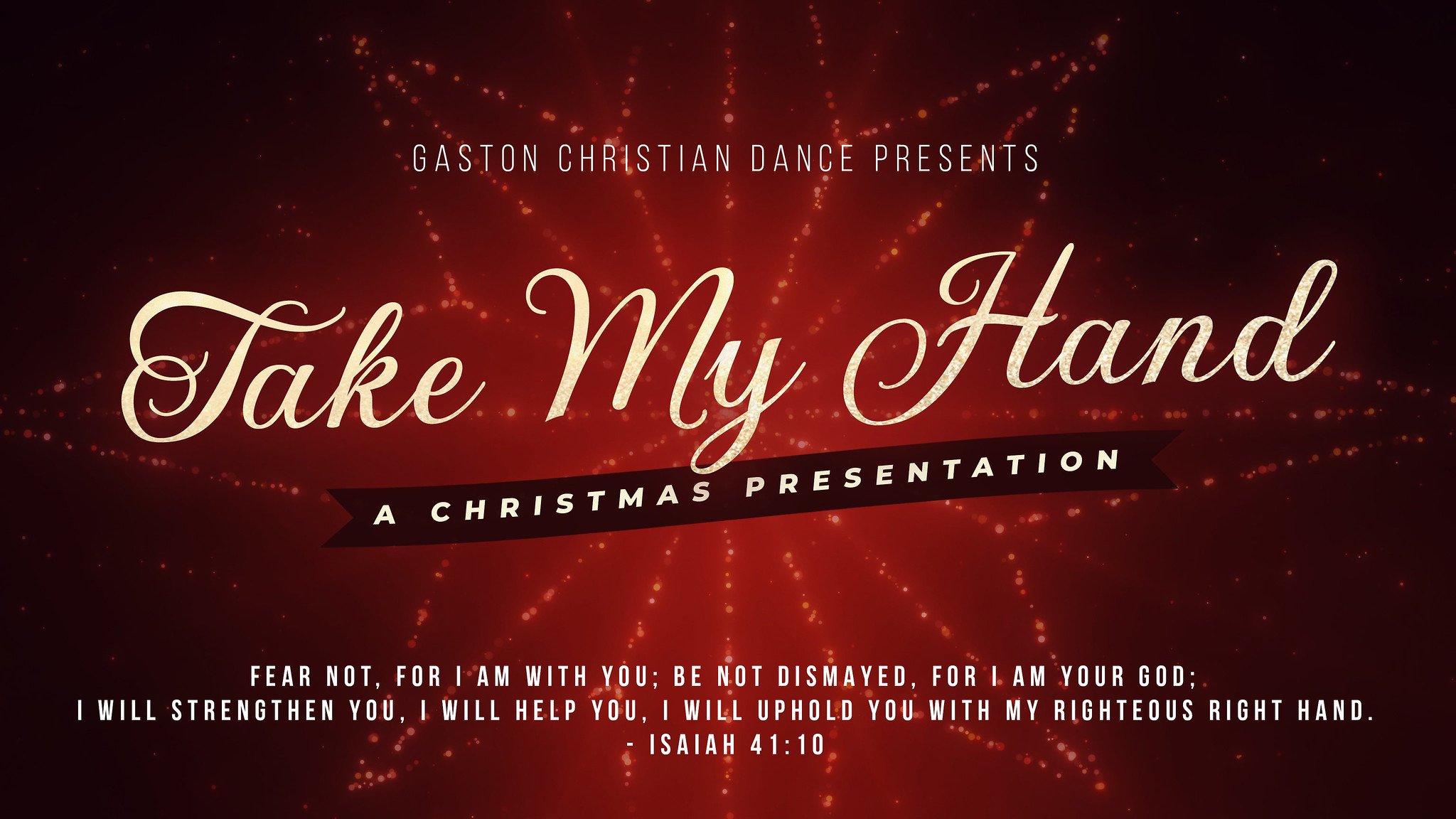The advertisement for the event features a rich burgundy background adorned with an intricate, glowing red outline of either a poinsettia or a star. At the very top, the text "Gaston Christian Dance Presents" is displayed in a small font. Centered in the middle of the star or poinsettia outline, the title "Take My Hand" stands out in gold, glittery cursive text. Just below the gold headline, a slightly wavy black banner bears the words "A Christmas Presentation" in elegant black text. At the bottom of the graphic, in white print, there is an inspirational Bible verse: "Fear not, for I am with you; be not dismayed, for I am your God. I will strengthen you, I will help you, I will uphold you with my righteous right hand. Isaiah 41:10." The overall design emanates a festive, starry ambiance, making it a captivating Christmas event notification that would be perfect for sharing on social media platforms like Facebook.